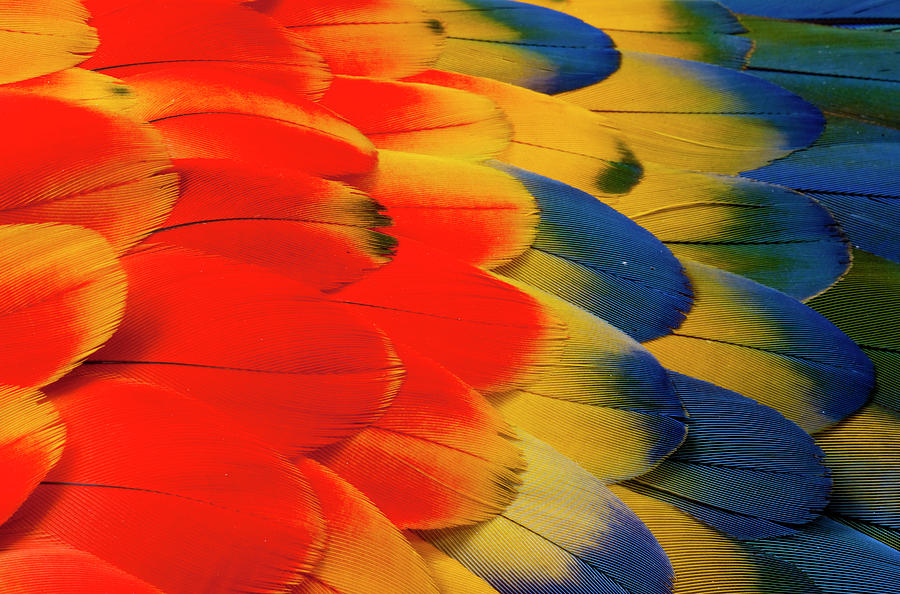This vibrant, close-up color photograph captures an elaborate and meticulously arranged display of parrot feathers. The feathers are organized in horizontal rows, transitioning through a vivid spectrum of colors. On the left, the feathers predominantly feature bright red centers with contrasting yellow edges, some with small black spots at the tips. Moving rightward, the feathers remain primarily red, with occasional touches of yellow and black. Further along, the red and yellow mixture intensifies, with several feathers showcasing more yellow than red. The arrangement continues with rows of feathers transitioning to striking blue and yellow—some starting yellow with blue tips, others mostly blue. The final visible row presents predominantly dark blue feathers, with hints of green-tipped feathers interspersed. This visually stunning array underscores the parrot's natural beauty, though the photograph itself remains unsigned and undated.